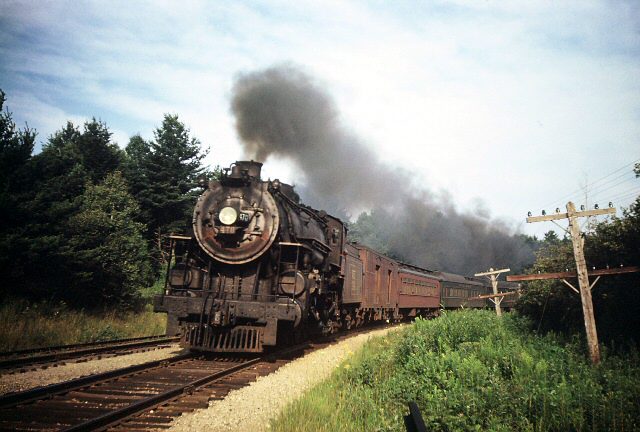The photograph captures a detailed scene of a vintage steam train, likely from the 1920s or earlier, set against a partly cloudy blue and white sky. This horizontally aligned image shows the black locomotive making its way around a curve, approaching from the right and moving towards the lower left corner of the frame. The front of the train, with its distinctive round face, central light, and large smokestack emitting dark gray smoke, dominates the foreground slightly to the left of center.

On the left side of the image, there's a line of coniferous trees standing tall, with patches of green and dry grass at their base. The two railroad tracks running through the scene are flanked by white gravel, with additional lush greenery and dense foliage on the right side of the tracks. There are brown wooden power line poles, supported by diagonal braces, that add character to the setting. These power poles seem somewhat slanted, possibly due to sinking into the ground, and are accompanied by large bushes and more trees in the background.

The train itself pulls a series of old-style passenger cars. The first few cars are reddish with yellow stripes, followed by darker gray or black cars. The train’s leading engine features a large horizontal cylinder, a rectangular vent with vertically aligned bars, and a possible standing area with handrails and ladders. The grain of the photograph suggests it might have been taken in the last 15 years, despite showcasing a train design from the early 20th century.